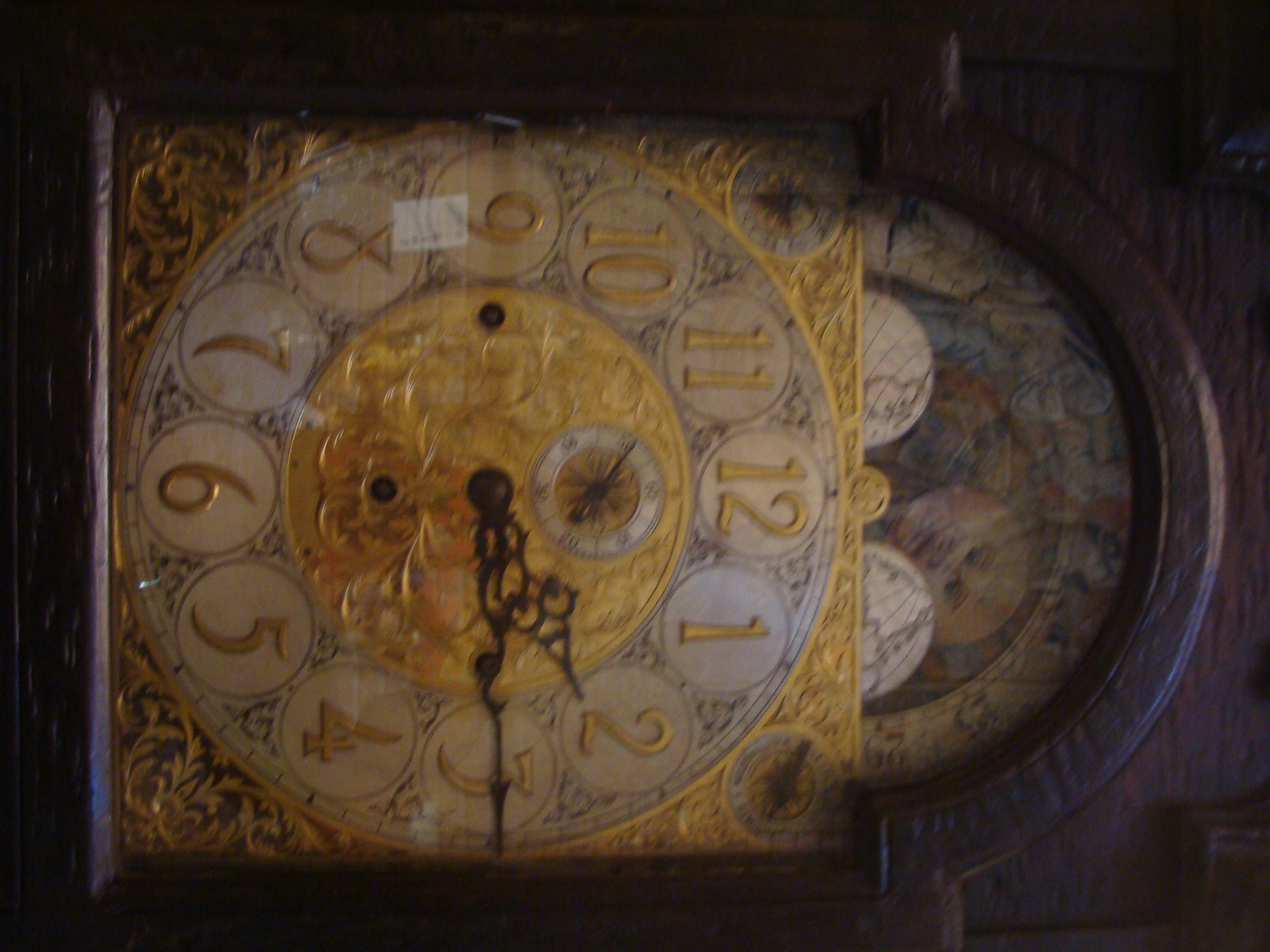The image depicts the intricately designed top section of a grandfather clock, but it is taken from a sideways perspective. The main clock face, which is gold, prominently showcases the time as quarter past two with its black hour and minute hands. Surrounding the clock face is a polished wooden frame, characteristic of traditional grandfather clocks. A celestial dial featuring a moon phase indicator runs horizontally below the clock face, tracking day and night cycles. Additionally, there are two smaller dials located at what would typically be the upper left and right corners, each equipped with tiny hands, likely serving as additional instrument indicators, possibly for measuring humidity or atmospheric pressure.